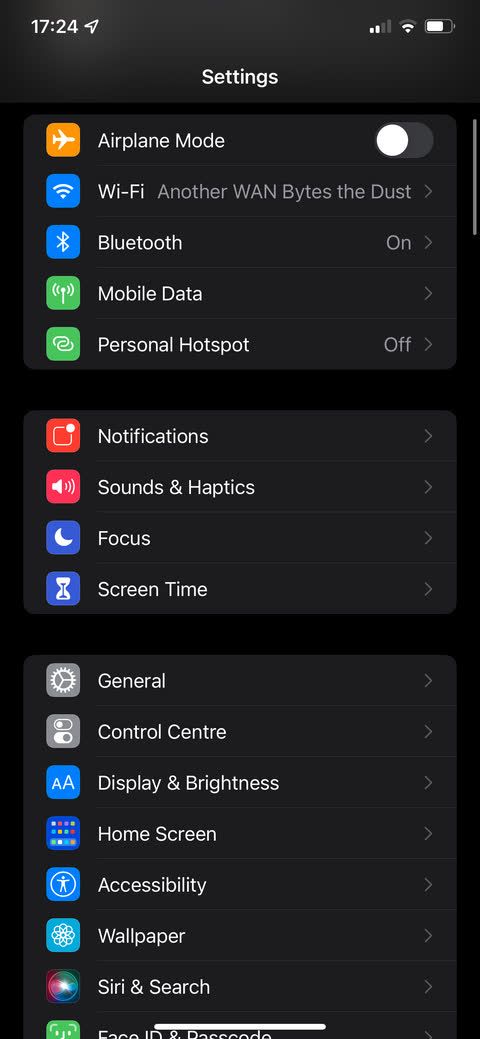A detailed screenshot of an iPhone settings menu displayed in dark mode. The background is black, and the settings list is in white text. In the upper left corner, the time is shown as 17:24, accompanied by a location icon. In the upper right corner, indicators for battery percentage, Wi-Fi signal strength, and cellular signal strength are visible. The title "Settings" appears centered at the top of the screen in white text.

The settings menu is divided into three distinct sections, each containing various options:

1. The first section includes:
   - **Airplane Mode**: Toggle switch to enable or disable.
   - **Wi-Fi**: Has a right-pointing arrow for further options.
   - **Bluetooth**: Has a right-pointing arrow for further options.
   - **Mobile Data**: Has a right-pointing arrow for further options.
   - **Personal Hotspot**: Has a right-pointing arrow for further options.

2. The second section includes:
   - **Notifications**: Has a right-pointing arrow for further options.
   - **Sounds & Haptics**: Has a right-pointing arrow for further options.
   - **Focus**: Has a right-pointing arrow for further options.
   - **Screen Time**: Has a right-pointing arrow for further options.

3. The third section also includes several options, similarly formatted with right-pointing arrows for additional settings, although these specific entries are not detailed in the provided description.